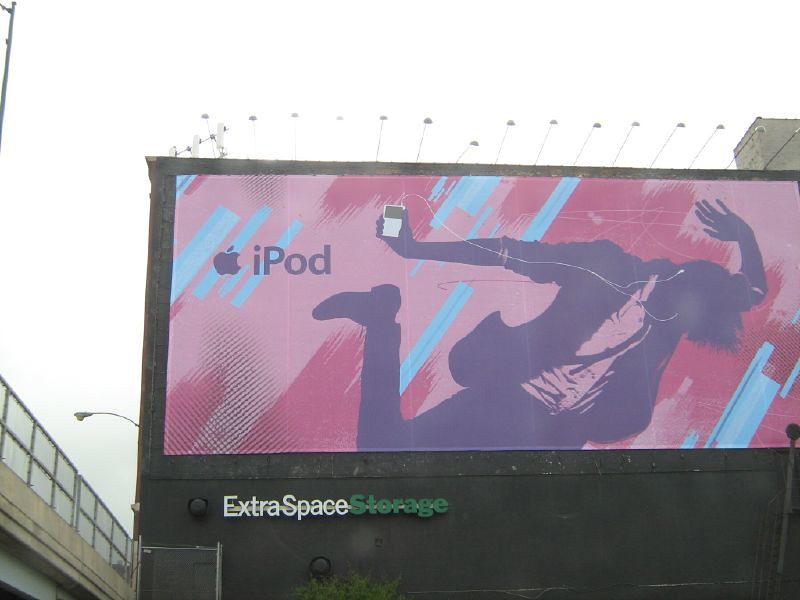The image depicts a large roadside billboard attached to the side of a black building, which has a beige concrete base and a chain-link fence running alongside it, possibly an underpass of a concrete bridge with fencing on the right-hand side of a walkway or a bridge. The top left corner of the image shows the upper part of a steel light pole. The building features a nameplate reading "Extra Space" in white letters and "Storage" in green letters at the bottom of the billboard. Above this nameplate is an advertisement showcasing an Apple iPod. The billboard has a vibrant pink, blue, and mauve background with diagonal stripes. It features the silhouette of a person dressed in a black blazer, white button-down shirt, thin tie, black pants, and shoes. The person is dancing, their right arm extended to the side, left arm bent behind their head, right leg kicked up, with white headphones leading from an iPod in their right hand to their ears. The person's head is bowed forward, with hair flung straight down, and the back of their blazer and tie are vividly animated, reflecting the dynamic movement. At the top of the billboard are branched lights meant to illuminate the advertisement, against a backdrop of clear sky with clouds.